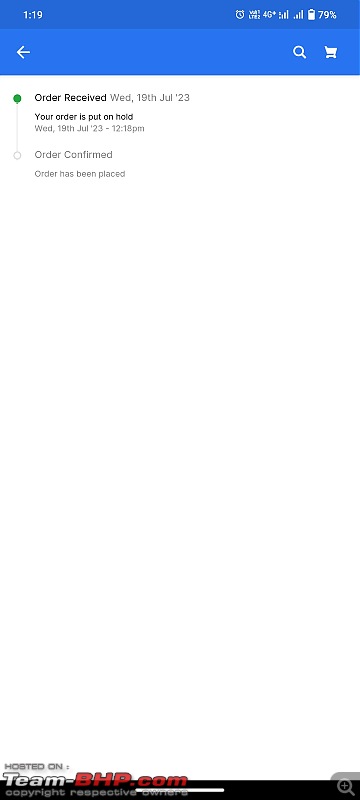This image is a screenshot of a mobile phone page, capturing a detailed view of an order status update. At the top, a dark blue header spans across the screen, featuring white icons on each end. Directly below this is a medium blue header with a white arrow pointing left on the left side and two white icons—a magnifying glass and a shopping cart—on the right side.

The main body of the page has a white background. In the top-left corner, there is a green circle, from which a vertical light gray line extends downward a short distance to a light gray outlined circle with a white fill. To the right of the green circle, small black text reads "Order received," accompanied by the light gray text "Wednesday, 19th, July 23."

Beneath this, aligned to the left, is a smaller line of black text stating, "Your order is put on hold." Just below, in light gray text, "Wednesday, 19th, July 23 - 12:18 PM" is displayed. Following a line break is light gray text reading "Order confirmed," and beneath another line break, smaller light gray text states, "Order has been placed."

At the bottom of the frame is an overlay with three lines. The top line, in all caps dark gray text, says "HOSTED ON:". Below this, italicized blocky text with a black outline reads "team-bhp.com," where "TEAM-" is in white and "bhp.com" is in red. The final line features light gray lowercase text indicating "copyright respective owners."